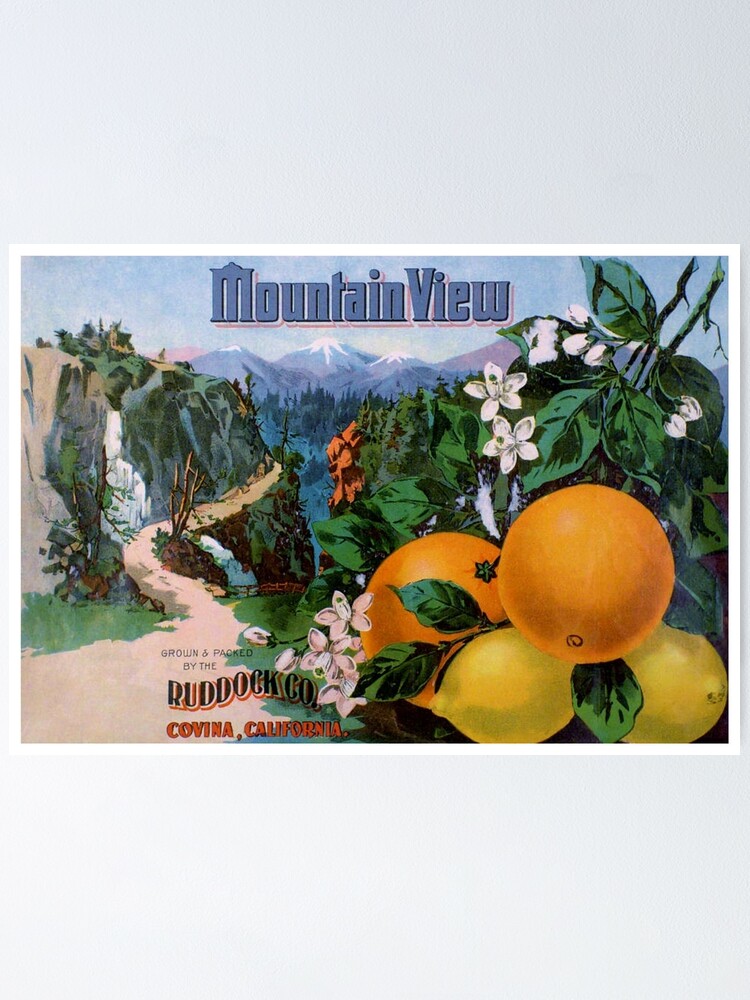The image depicts a vintage-style postcard from Colvin, California, measuring approximately six inches high by four inches wide, with a background gradient transitioning from steel gray at the top to pale light gray at the bottom. Dominating the top section in bold, fat blue letters outlined in pink and white, the text "Mountain View" prominently stands out. The lower right half of the image showcases vibrant oranges and lemons adorned with green leaves and delicate white flowers, set against a faintly visible tree. To the left, a dirt trail winds up a hillside, leading towards a picturesque landscape featuring snow-capped mountains and a forest beneath a clear blue sky. Centrally positioned just below the middle, there is an inscription that reads, "Grown and packed by the Ruddick Co., Ruddick Company, Covina, California." The postcard intricately merges vibrant shades of orange, yellow, green, blue, beige, white, and purplish hues, creating a nostalgic and colorful representation of the region’s natural beauty.